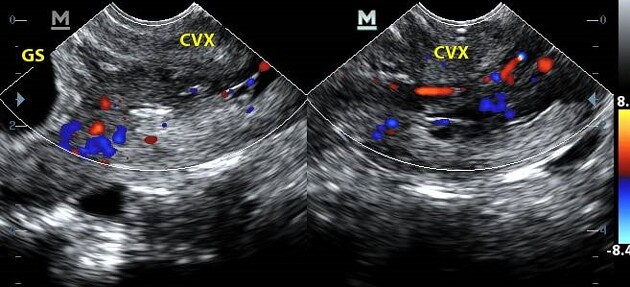This image features two separate ultrasound scans on a black background. The scan on the left displays a quarter-circle area containing the yellow letters "GS" on the far left and "CVX" towards the right, amidst a sea of speckled white dots and blurs. Additionally, red and blue speckles are distributed across this image. The scan on the right mirrors this layout with "CVX" at its center and a color scale ranging from yellow to blue on the extreme right. Both scans incorporate red and blue speckles, indicative of color Doppler technology. These images include the letter "M" in the top left corner, suggesting measurement or scale components, and the color scale runs from minus 8.4 to 8.0, further adding to the detailed diagnostic information presented.